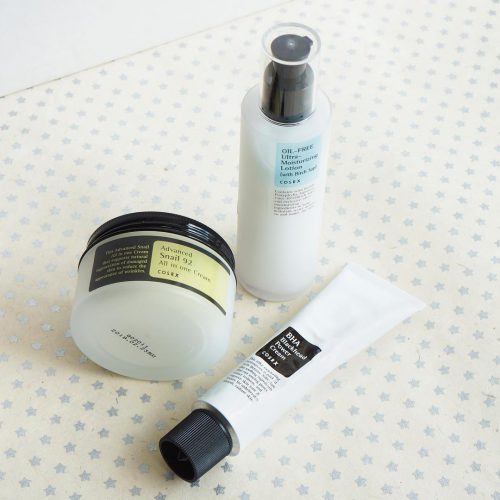Photographed on a whitish-yellow tabletop adorned with a silver star pattern, this image displays an assortment of skincare products. The background features a white wall, and the photo is taken from a slight upward angle, offering a detailed yet dynamic view of the items. Central to the composition is a circular jar with a black metal lid, partially opaque, and made of clear material. It features a black label with yellow text that reads, "Advanced Snail 92, All-in-One Cream." Adjacent to this jar is a compact spray bottle, distinguished by its white cylindrical shape and a black cap, labeled "Oil-Free Ultra-Moisturizing Lotion." Completing the trio is a white tube with a black label bearing the inscription "BHA Blackhead Power Cream," topped with a matching black cap.